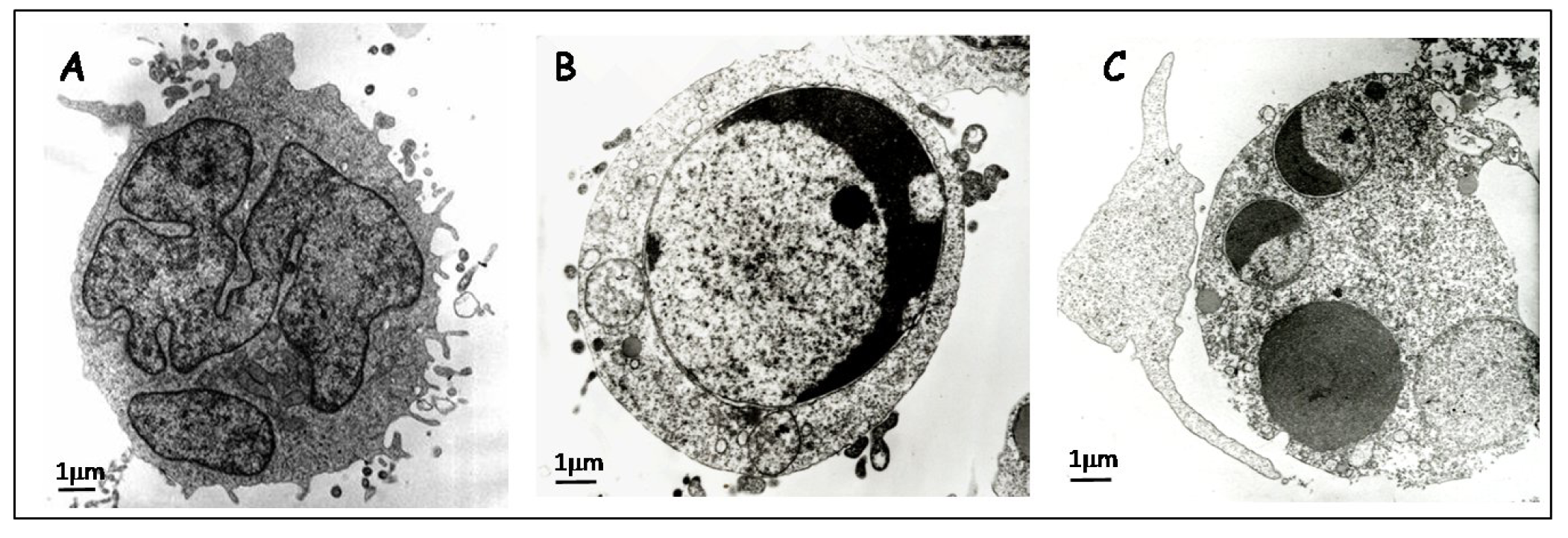This composite image comprises three highly magnified black-and-white electron micrographs labeled A, B, and C, each showing a distinct cell, with a scale bar indicating one micron. 

Image A features a somewhat circular cell with irregular, rocky borders and dense cytoplasm filled with numerous small, black specks and splotches. The interior houses various irregular black-outlined shapes, possibly representing the nucleus or other dense bodies.

Image B displays a larger, almost spherical cell characterized by a prominent central inclusion, giving it a crater-like appearance with a darker, shadowed crescent area that suggests depth. The cell boundary here is well-defined.

Image C presents an oval-shaped cell with multiple large circular areas inside, potentially vacuoles or other organelles, along with some craggy textures and darker gray circles overlaying a lighter gray background.

All images share a common label in the lower-left corner: "1 μm," indicating a scale of one micron, crucial for understanding the magnification level. The images are detailed yet complex, evoking the feel of textbook illustrations aimed at teaching cellular structures.